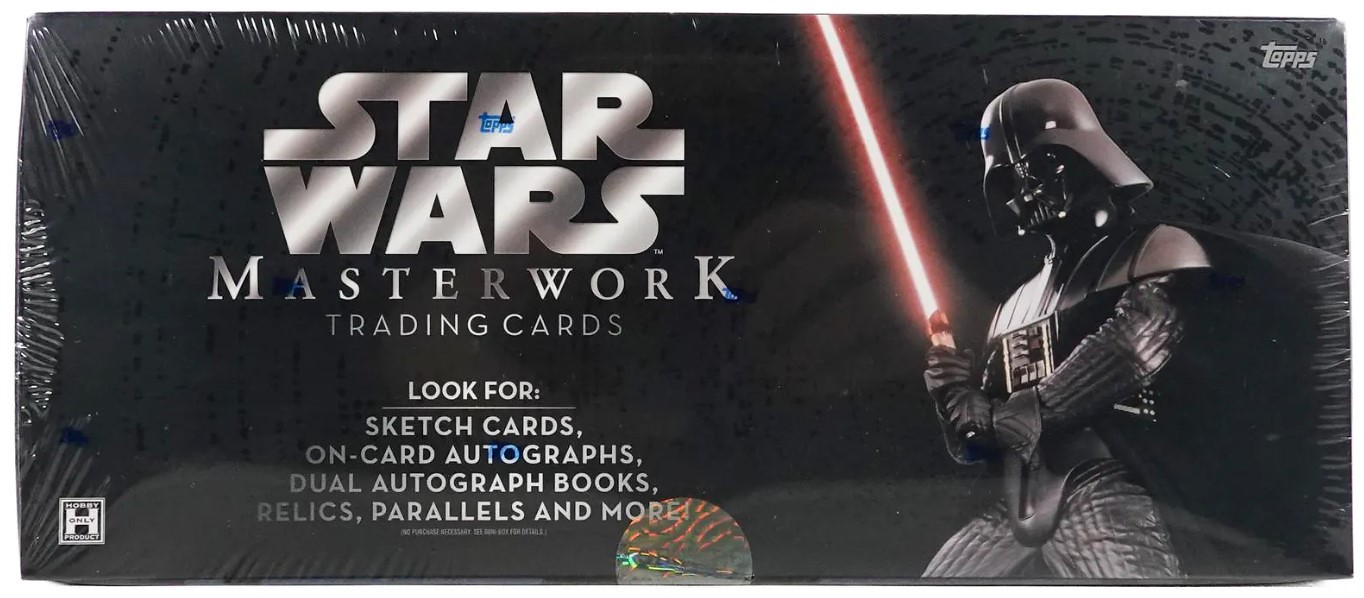The image prominently features a rectangular, all-black package of Star Wars Masterwork Trading Cards, completely filling the frame with no visible background. In the center, white and gray lettering announces "Star Wars" with "Masterwork Trading Cards" beneath it. Dominating the right side of the box is an illustration of a Star Wars character in a shiny black helmet and cape, gripping a brightly lit lightsaber. The lower part of the package details the potential contents in white text, including sketch cards, on-card autographs, dual autograph books, relics, parallels, and more. The palette of the package includes colors like black, white, gray, blue, pink, orange, and green, giving it a striking and collectible allure. This box, similar to something found in a toy store, emphasizes its premium nature and collectible appeal.